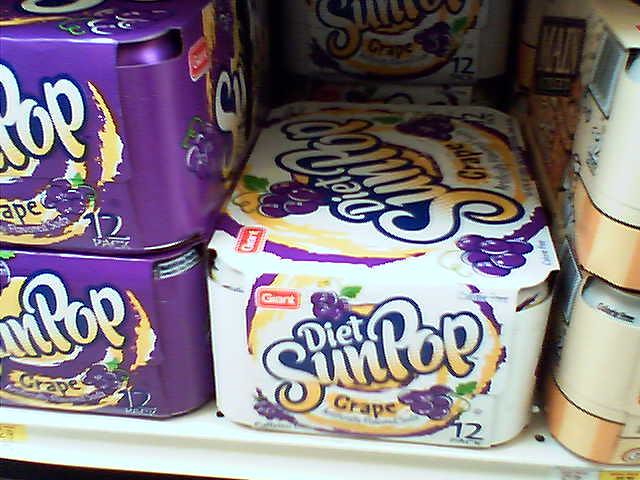In the image, we see a close-up of a single off-white modular shelf inside a store, likely a grocery or convenience store, displaying various packs of soda. On the left side of the shelf, there are two 12-packs of Sun Pop Grape soda in purple packaging with white lettering that prominently displays "Pop" and "Grape," along with an image of grapes. In the center of the shelf, there's a single 12-pack of Diet Sun Pop Grape, featuring white cardboard packaging adorned with whimsical lettering, purple grape imagery, and a hint of gold and yellow at the top. This Diet variety is clearly marked and is partially stacked in front of two more packs of the same soda behind it. On the right side of the shelf, there are two more 12-packs in tan sleeves, though their exact contents are not visible. The entire arrangement gives a neat, compact view of the Sun Pop soda products, highlighting both the regular and diet grape flavors.